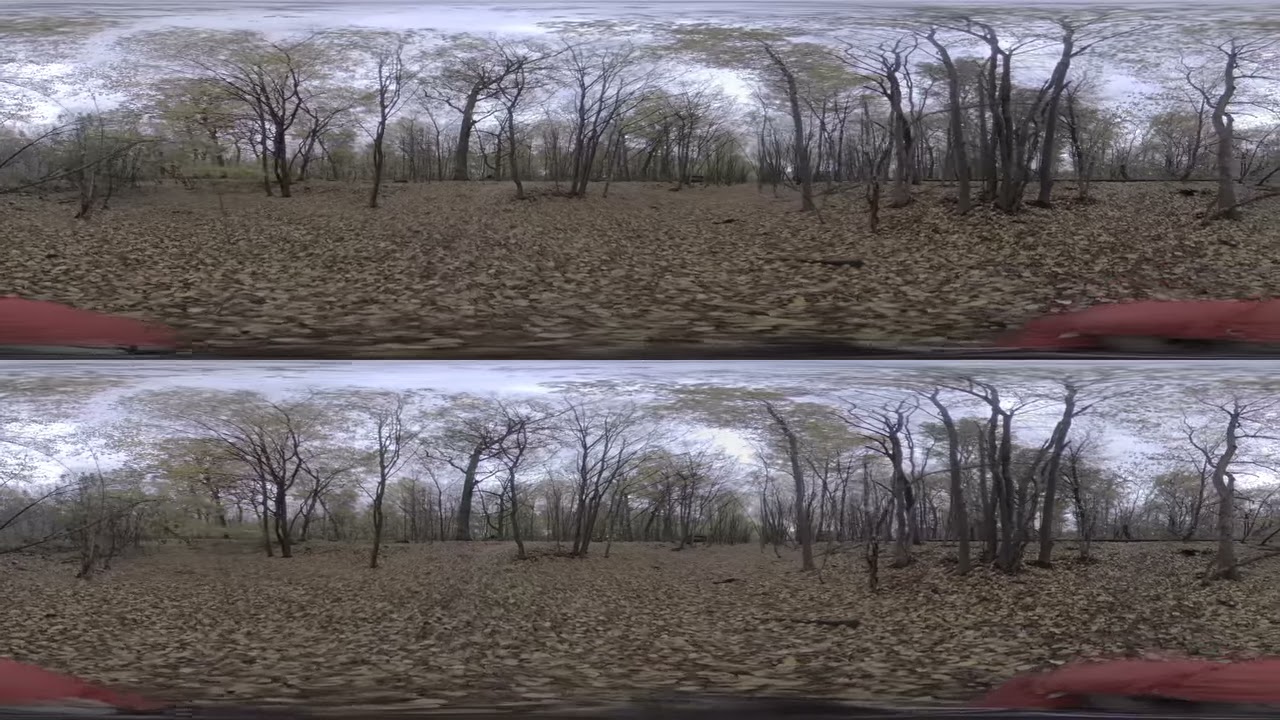The image features two identical and elongated panoramic pictures, one placed on top of the other, both depicting a wintery forest scene that appears blurred and out of focus, possibly due to motion when the photo was taken. The trees are gnarled and bare, with a thick layer of brown, dry leaves covering the forest floor. Scattered pieces of wood add to the desolate appearance. The overcast, grayish-white sky enhances the wintry feel, while mysterious red streaks appear on the bottom left and right corners of the image. Despite the blur and elongation, the overall scene captures the stark, barren beauty of the forest in late autumn or early winter.